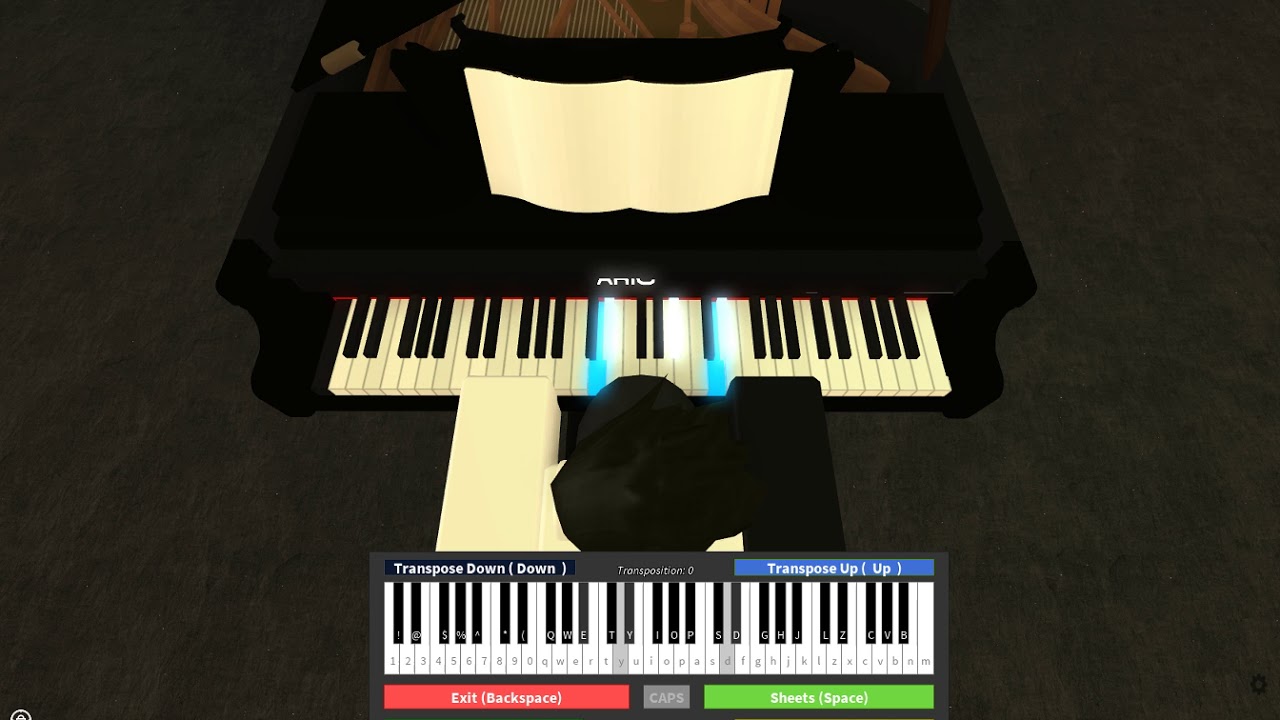In the digital image, likely viewed on a computer screen or tablet, the primary focus is on two keyboards presented against a very dark gray background. The lower keyboard resembles a typical QWERTY keyboard, with each white key labeled with lowercase letters, and black keys labeled with uppercase letters or symbols. Notably, the bottom of this keyboard features "EXIT (BACKSPACE)" in red, "CAPS" in gray, and "SHEETS (SPACE)" in green. Above this keyboard is an animated piano with off-white and black keys, devoid of any labels. Above the piano sits a white sheet of music on a stand, with the piano's internal strings visible, suggesting a detailed, interactive digital representation. Two keys on this piano are highlighted in blue. Additional on-screen labels include "Transpose Down" and "Transpose Up" in blue. A character wearing a hat suggests an over-the-shoulder view, reading the music. The color palette includes shades of brown, black, off-white, blue, red, and green, consistent with a video game or educational software interface.